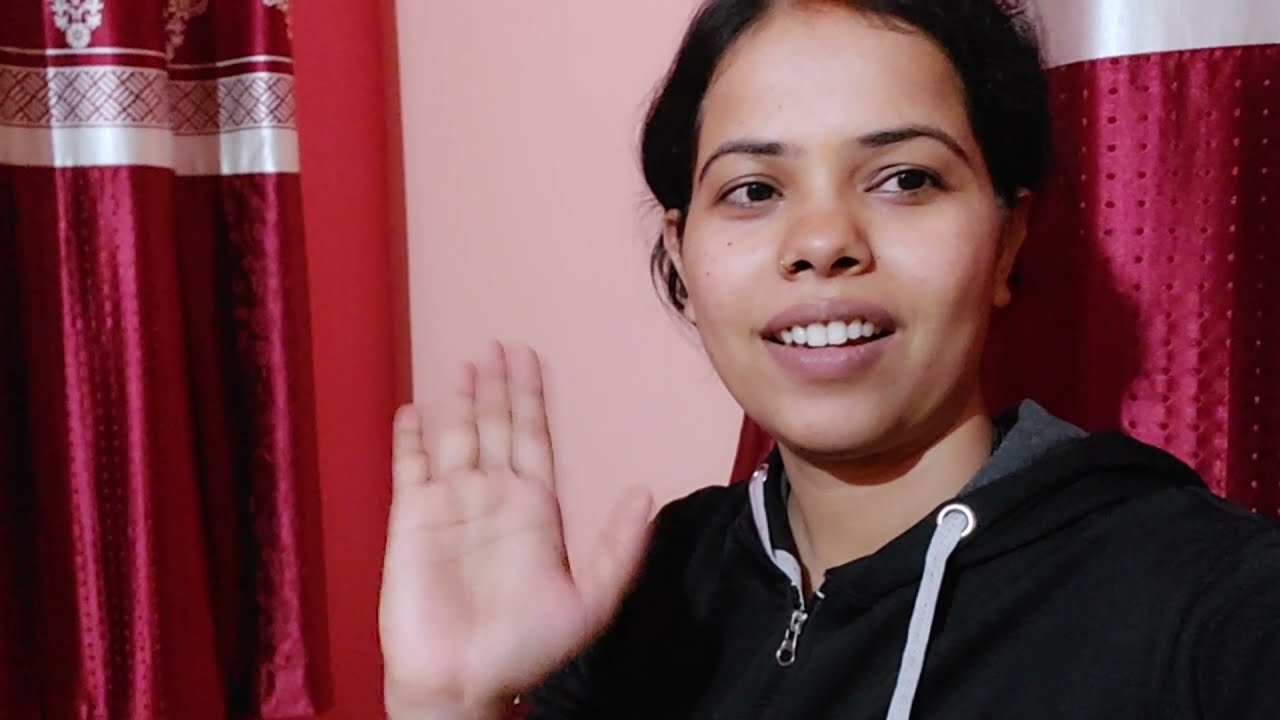The photograph features a young woman positioned slightly to the right of the center of the image, with her face turned towards the camera but her dark brown eyes looking to the right, her left. She has an olive complexion, dark hair pulled back behind her ears, and expressive features including full lips with a hint of pink gloss, a nose ring on her wider nose, and dark eyebrows. She’s wearing a black hoodie with a zipper and white drawstrings, and her right hand is raised, palm towards the camera, as if she is taking an oath or waving. A light smile graces her face, revealing the upper row of her teeth. The background consists of a light pink wall adorned with dark reddish-pink curtains featuring white patterns and small embossed dots. The curtains are positioned on both the left and right sides of the image, framing her figure.